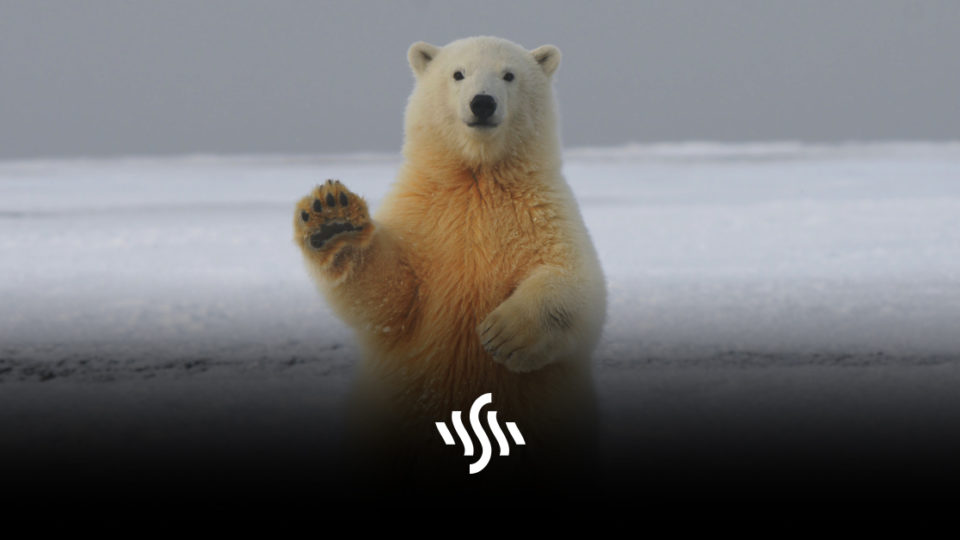In this picture, a polar bear stands against a snowy, tundra-like backdrop with a light gray, cloudy sky overhead. The bear, more of a cream color than the pure white often associated with polar bears, has its right paw (left side from the viewer's perspective) held up in a wave-like fashion while the other paw rests on its chest, giving the impression that it's greeting the viewer. The polar bear's underbelly has a noticeable golden or even brownish tint. The image gradually fades to black at the bottom, creating a stark contrast with the snow. Positioned around the bear's belly area, where a belly button might be, is a logo consisting of an 'S' accompanied by two diagonal white lines on each side.